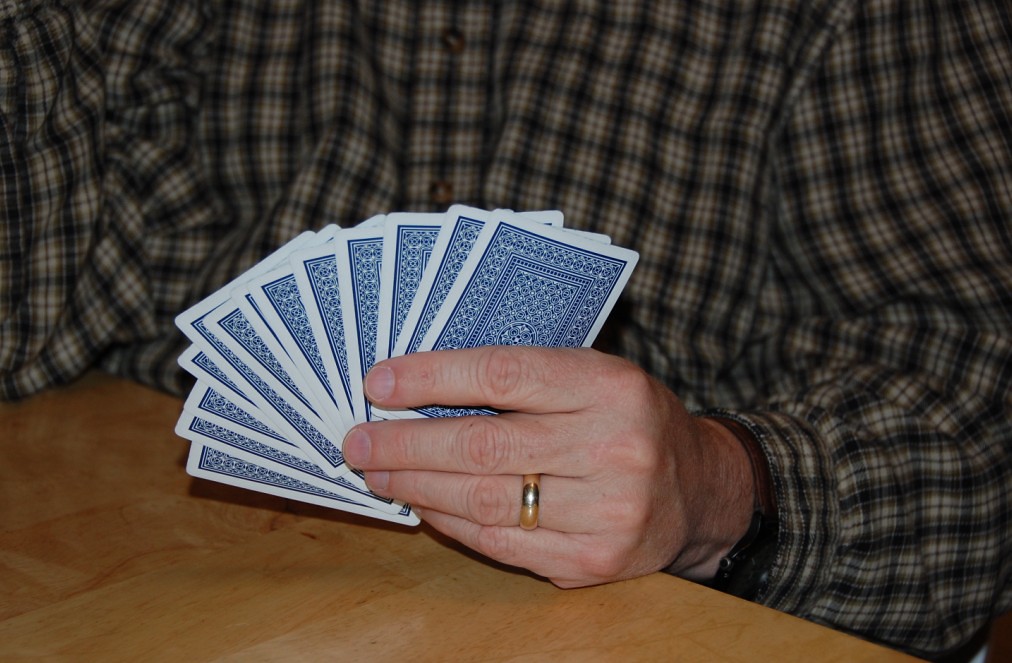In the photograph, a person's left hand is prominently featured playing cards, with the rest of their body out of view. The hand is holding approximately ten blue cards, each adorned with an intricate, ornate pattern on the back, nestled closely to the fingertips, ensuring only the back design of the cards is visible. The individual is wearing a gold wedding band on their left ring finger. The hand is resting on a wooden table. The person is dressed in a checkered plaid shirt featuring a tan background with dark green, black, red, and possibly orange lines.